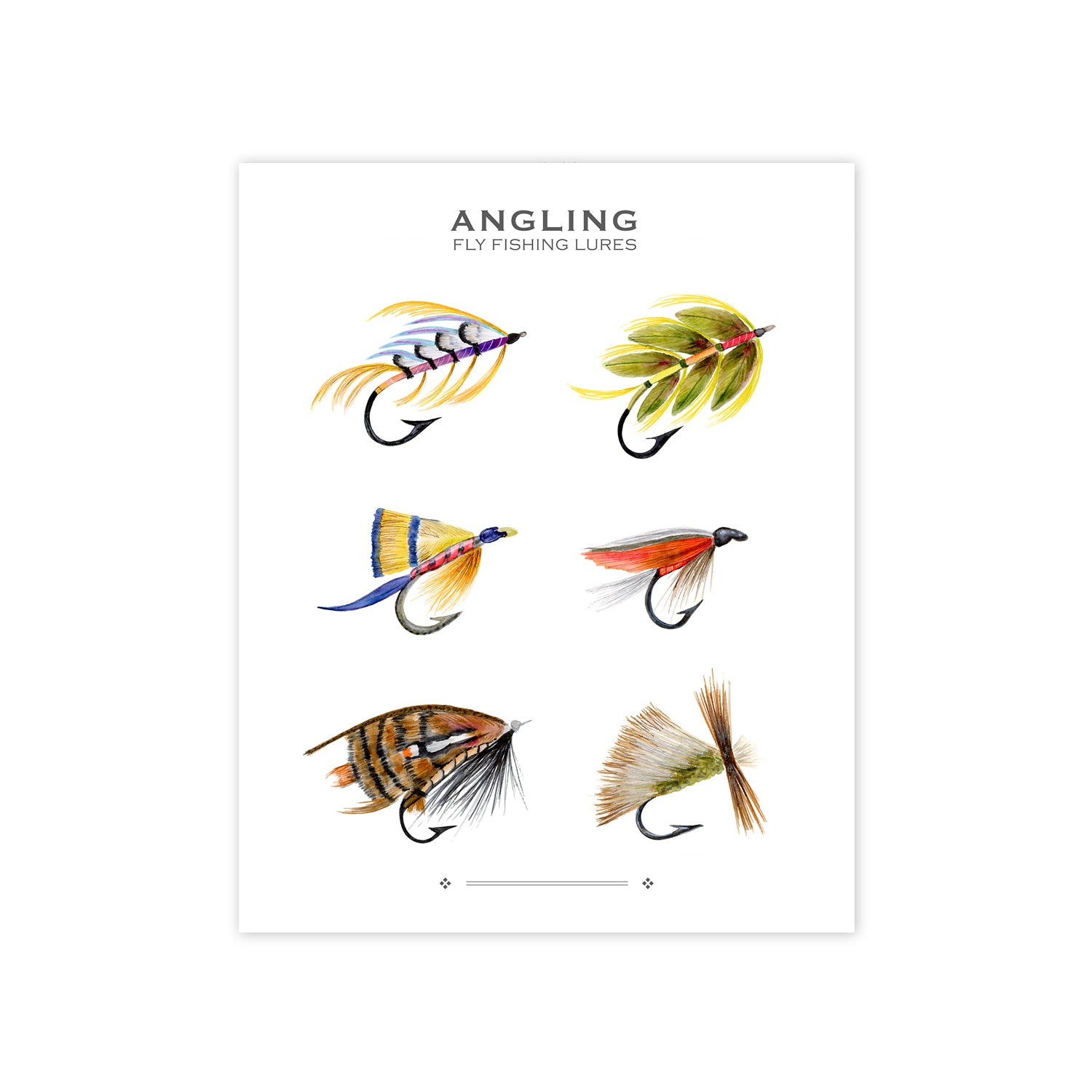The image is an 8 by 10 illustration with a white background and a gray-bordered rectangular frame with a subtle drop shadow. At the top, in bold dark gray uppercase letters, are the words "ANGLING," followed by "Fly Fishing Lures." Below the title, there are six fly fishing lures arranged in three rows and two columns. Each lure's hook points towards the upper right corner.

In the top row:
- The left lure has black feathers with yellow and purple accents.
- The right lure features green leaf-like projections with a black hook.

In the middle row:
- The left lure resembles a yellow and blue broom shape.
- The right lure is reddish with white and gray colors, giving a bird-like appearance.

In the bottom row:
- The left lure has black stripes and orange accents, resembling a small fish.
- The right lure is brown and white with feathered extensions, reminiscent of a butterfly wing or cat whiskers.

At the bottom of the image, there's a decorative line with diamond shapes on either side.